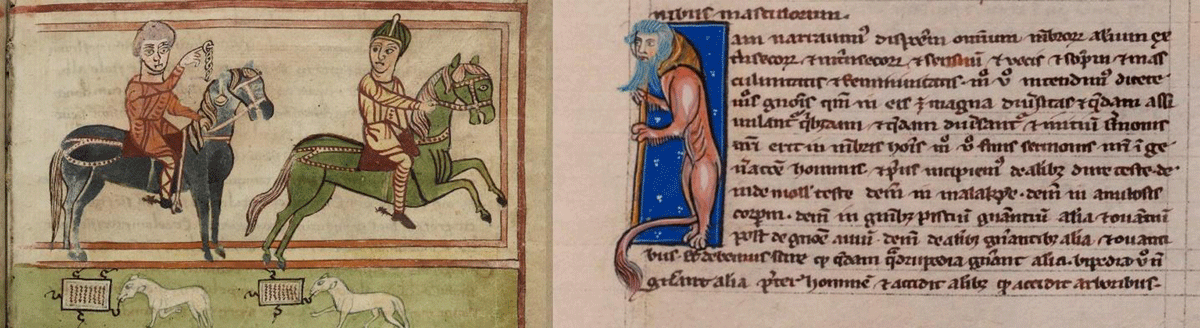The image depicts a long horizontal illustration, resembling an illuminated medieval manuscript. On the left side, two men on horseback are shown in a simplified, two-dimensional style. The man on the left rides a black galloping horse and dons an orange outfit, while the man on the right is on a stationary green horse, wearing a tan-colored outfit and looking back. He holds a spiral chain-like item hooked over his finger. Below them, a couple of white dogs are depicted chewing on manuscripts, adding a touch of complexity to the scene.

In the middle and right sections of the image, there is a large block of highly ornamental text written in an elaborate calligraphic script, possibly in French or Latin. Adjacent to the text, on the left side of it, stands a humanoid figure with the body of a lion and the face of a human, leaning on a pole against a deep blue background. This vertical strip beside the text enhances the artistic intricacy of the manuscript, suggesting it might be part of a medieval novel or historical document. The figures on horseback and their well-decorated attire, combined with the unusual creatures and elaborate script, create an impression of wealth and mystery, capturing a moment from a richly illustrated historical narrative.